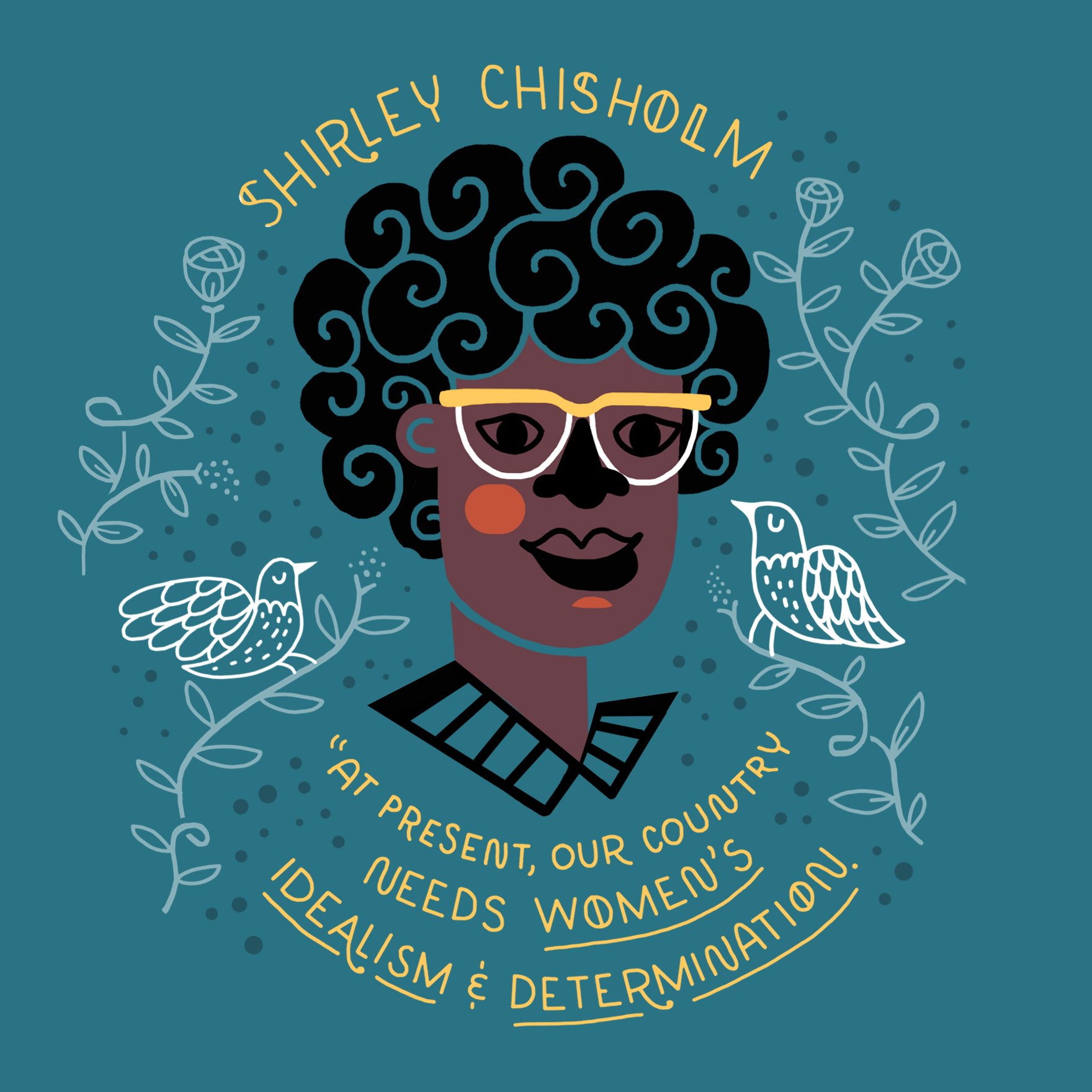This detailed modern art illustration features a prominent portrait of activist Shirley Chisholm at its center. She is depicted from the top of her head to around mid-neck, set against a dark aqua background with graphic design elements. The portrait showcases Shirley's curly black hair accentuated with blue curves, dark skin with a prominent orange dot on her cheek, and striking yellow-framed eyeglasses. She is dressed in a collared shirt featuring blue and black hues. 

Overlaying the image are two arcs of text in bright yellow. The top arc presents her name, "Shirley Chisholm," while the bottom arc quotes, "At present, our country needs women’s idealism and determination," with "women's idealism and determination" notably underscored. Flanking her portrait on both sides are white-outlined illustrations of birds facing inward towards her. Additionally, flourishes of rosebuds on vines, drawn in a delicate white, surround her face. This piece is a vibrant and detailed color illustration, blending modern art with thoughtful typography and graphic elements.